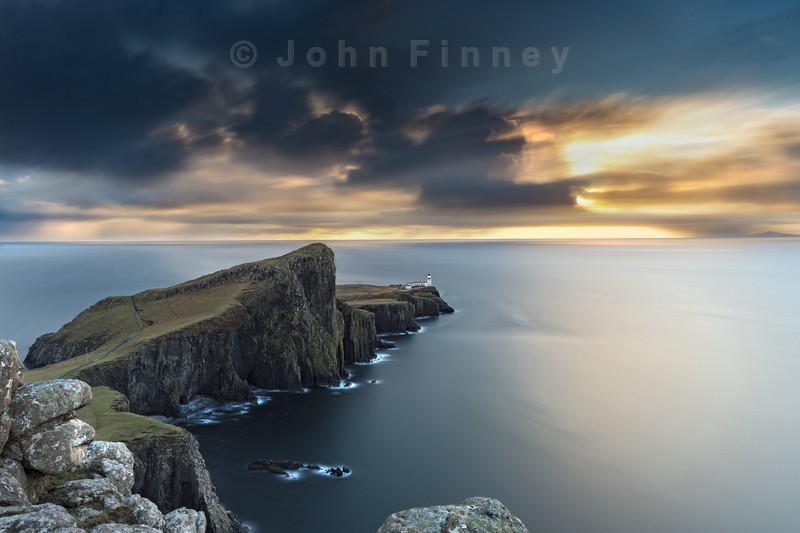The photo captures a tranquil ocean scene at sunset, with the horizon dominated by a dramatic cloudscape. At the top of the image, dark bluish-gray clouds blend into white and orange streaks with beams of sunlight piercing through. The water below appears almost silky smooth, perhaps due to a time-lapse effect, and glows with a blue hue tinged by the sunset's yellow light. The ocean, a dark bluish gray, is mostly calm except for a few waves crashing against a large, jagged cliffside that juts out from the lower left of the frame into the middle of the image. This cliffside, composed of tall, gray rocky walls, is adorned with patches of green moss and thin grass at the top. Some parts of the cliff extend into the water, where scattered rocks emerge from the sea. In the distance, a white lighthouse stands near the shore. The image is signed "Copyright John Finney" in light blue text at the top center, and rocky formations dominate the foreground.